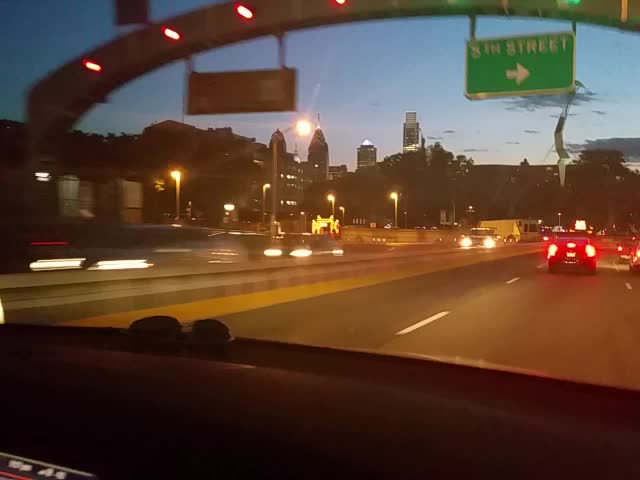The image captures a nighttime freeway scene from the perspective of a car's dashboard. The road, illuminated by the vehicle's headlights, stretches ahead. Distinctive dashed white lines delineate the lanes of the black asphalt. A black car is positioned in the center lane, its red taillights glowing brightly. Overhead, the sky is a deep, starless blue, with several green highway signs indicating street names, one specifically pointing to the right, hanging from an archway. 

Stark lights dangle across the scene, enhancing the contrast between the dark road and the illuminated surroundings. A gray sign is visible on the left, helping to guide drivers. In the distant background, a city skyline stands tall, with numerous skyscrapers, their windows aglow, adding a sense of bustling urban life. The freeway is divided by a gray median; on the opposite side, there are cars with their headlights facing forward, adding to the movement and energy of the scene.